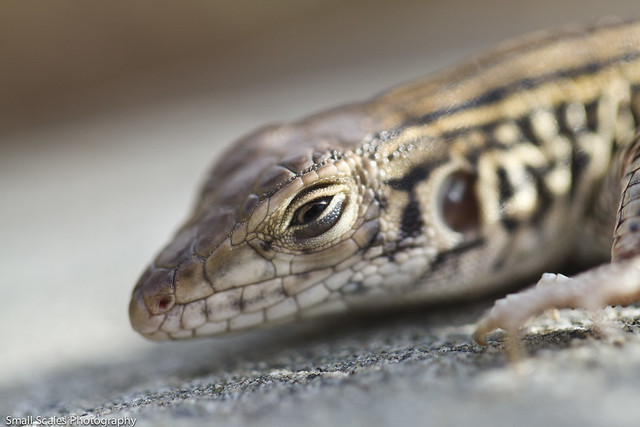The image captures a detailed close-up of a lizard in its natural environment during daytime, as indicated by the overall brightness. Positioned on a surface composed of grayish gravel or sand, the foreground features a mixture of brownish-tan hues that blend with the background's blurred-out shades of gray and brown. The lizard’s scaly head, slightly blurred at the top, brings out intricacies like its brown eyes, nostril, and a lengthy mouth. The lizard exhibits a pattern that combines dark brown, light brown, cream, and orange tones, with subtle touches of beige and tan. There appears to be a hole on the side of its head, likely its ear, adding to the detailed anatomy of the reptile. The image effectively focuses on the reptile, highlighting its texture and coloration against a naturally muted backdrop.